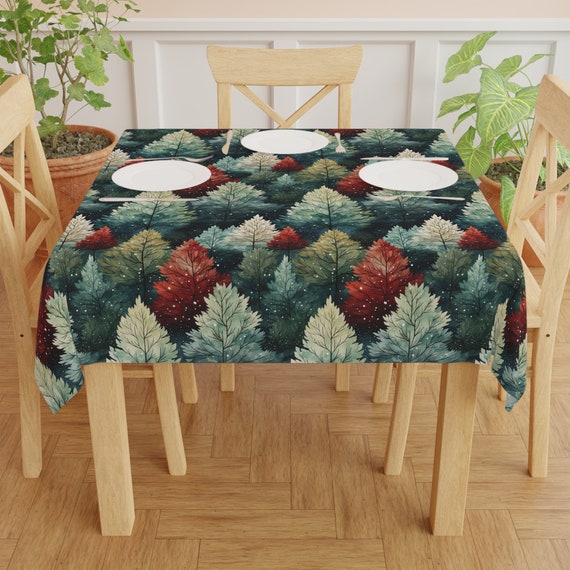A cozy square table is surrounded by three wooden chairs, all crafted from very light-colored wood. The table is adorned with a festive green tablecloth featuring an array of fir tree prints in shades of light green, red, and dark green. Each of the three place settings consists of a white plate, a fork, and a knife, neatly arranged on the table. The floor beneath is made of wooden panels laid in a distinctive zigzag pattern, adding character to the setting. Behind the table, two potted plants in clay pots contribute a touch of greenery to the scene. A glimpse of white wainscoting on a cream-colored wall adds an elegant backdrop, completing the inviting atmosphere.